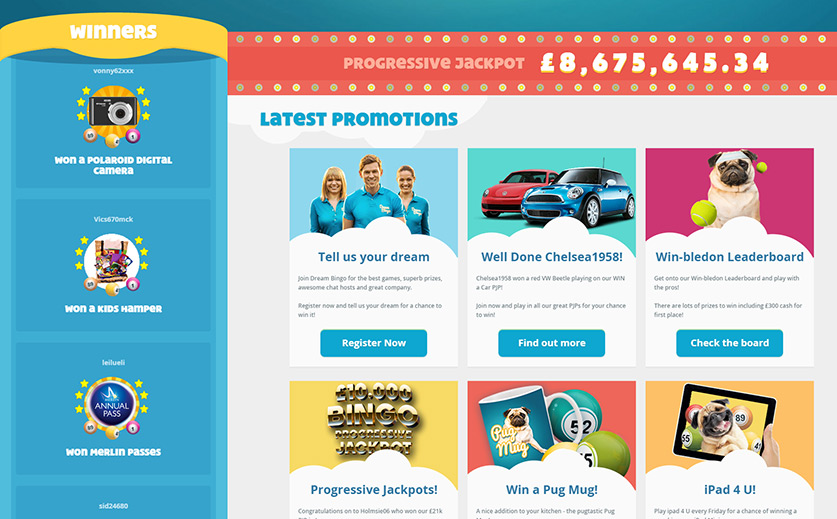"In this image, we see the winners of various prizes standing proudly. User 62XXX clinched a Polaroid digital camera, while user vix670 took home a delightful kid's hamper. Additionally, user leilueli achieved a remarkable feat by winning the Merlin Pass Progressive Jackpot, amounting to an astonishing £8,675,645.34. Congratulations are also in order for Chelsea1958, who topped the leaderboard and earned a Pogmog iPad through the 'Tell Us Your Dream' promotion. Well done to all the winners!"